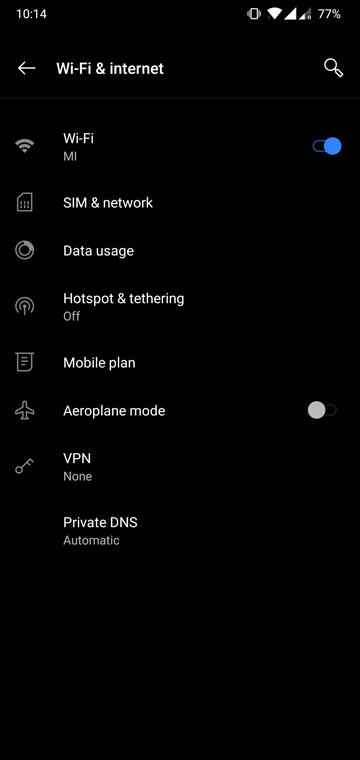This is a detailed screenshot from a smartphone screen with an entirely black background. At the top left corner, the time is displayed as "10:14", with no indication of a.m. or p.m. On the top right corner, the battery level is shown at 77%. Directly below, there is a white left-pointing arrow with the text "Wi-Fi and Internet" next to it. To the right of this text, a small magnifying glass icon is visible. 

Following a small gap, the Wi-Fi icon is shown, labeled "Wi-Fi mi" with a blue toggle switch next to it that enables the Wi-Fi feature. Below this, the words "SIM and network" appear.

Further down, the caption "Data usage" is visible with a toggle switch to the left. Adjacent to it, "Hotspot and tethering" is listed, which currently shows as turned off.

Below this section, "Mobile plan" is mentioned, followed by a drawing of an airplane icon with "Aeroplane mode" written next to it. This feature also has a white toggle switch beside it, indicating it is currently turned off.

In the next row, an icon resembling a key is observed, next to the word "VPN," which shows as "None" directly beneath it. Lastly, "Private DNS" is set to "Automatic." 

The screenshot ends with the bottom portion of the screen entirely black.